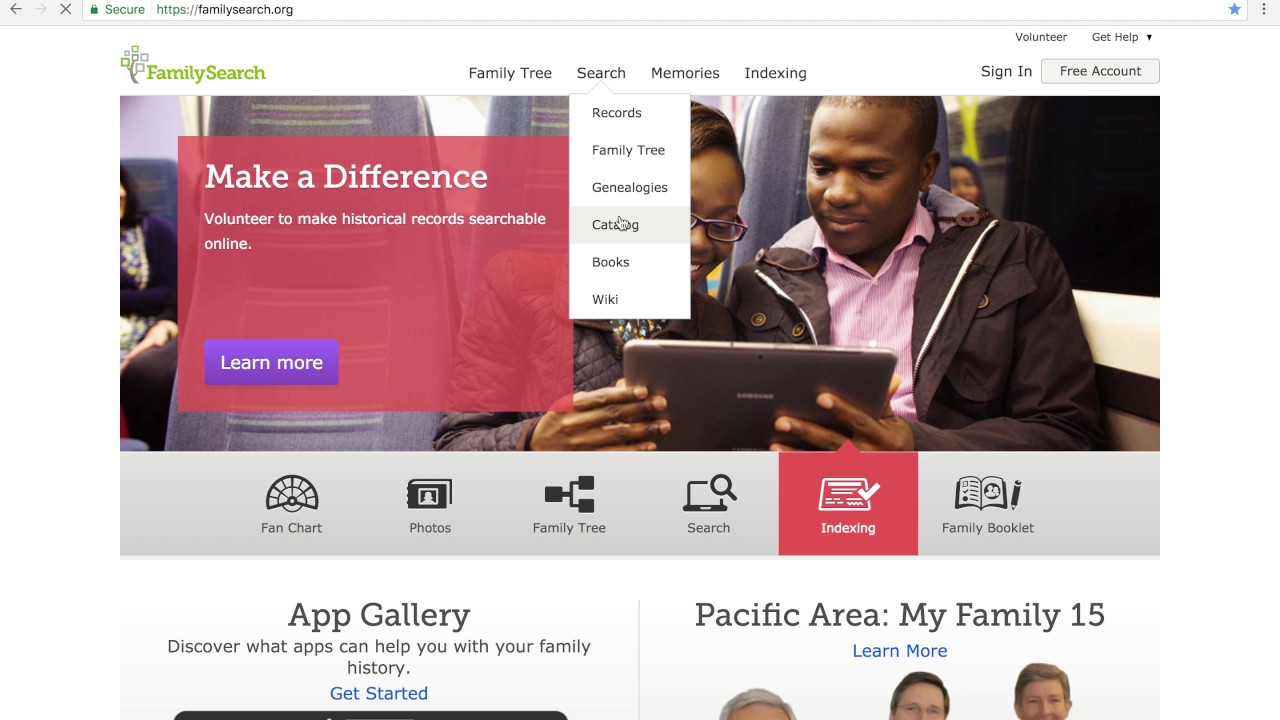Screenshot of the FamilySearch.org website:

At the top of the browser window is the URL bar, displaying "familysearch.org." The user has bookmarked this website, indicated by the filled star icon on the right-hand side of the URL bar.

Below the URL bar, the webpage header features the FamilySearch logo on the left, which consists of green lettering with "FamilySearch" next to a tree icon. The top navigation menu offers several drop-down options: "Family Tree," "Search," "Memories," and "Indexing." The user has hovered over the "Search" option, revealing additional clickable sub-options: "Records," "Family Tree," "Genealogies," "Catalog," "Books," and "Wiki." The cursor is specifically positioned over the "Catalog" sub-option.

On the right side of the header are buttons for "Sign In" and "Create a Free Account."

The main content area of the website displays a large, prominent image featuring two African-American individuals smiling and looking at a tablet. Adjacent to this image is text that reads, "Make a Difference. Volunteer to make historical records searchable online." Below this message, a pink translucent text box contains a purple button labeled "Learn More."

Further down, the website presents a series of icons with captions: "Fan Chart," "Photos," "Family Tree," "Search," "Indexing," and "Family Booklet."